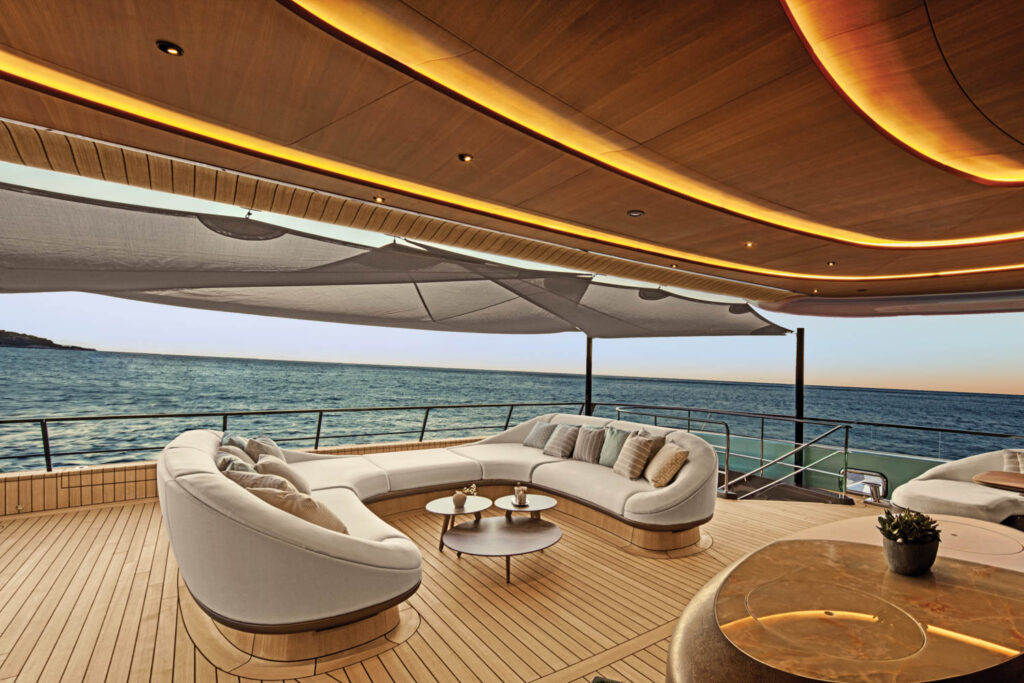This image captures the elegant and serene sitting area of a yacht's deck. The scene is framed by a C-shaped, cream-colored couch fitted with numerous striped throw pillows in shades of yellow, green, and gray. This couch is positioned on a curved wooden platform and is accompanied by a nested coffee table set, which includes one large circular table and two smaller, taller tables, each holding decorative items. The teak wood decking complements the design, and a wooden ceiling with recessed C-shaped lighting adds a warm ambiance. A small potted plant sits atop a marble countertop on the right side of the image, next to another matching, two-seater couch. Overhead, a netted sunshade offers protection from the sun. In the background, calm blue waters stretch out to the horizon, under a light blue sky, with a tiny piece of land visible on the left side. A metal fence encircles the area, adding a touch of security and sophistication.